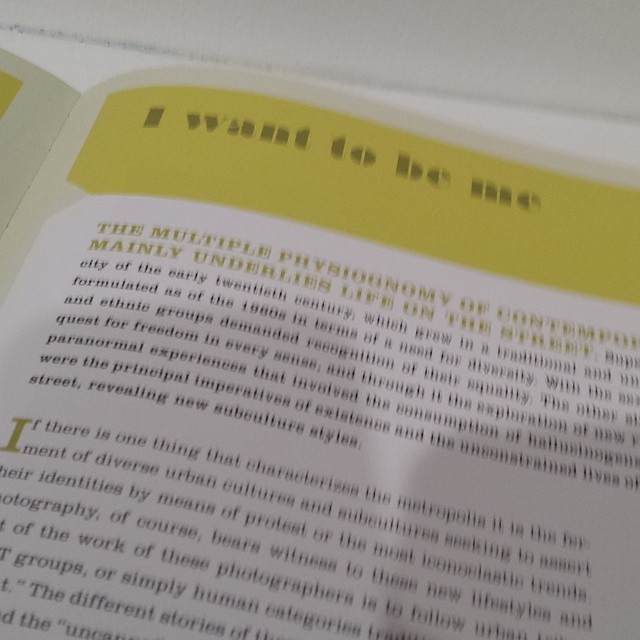The image depicts a slightly blurred photograph of an open book or magazine, with the focus on the right-hand page. The left page is partially visible at the edge of the frame. Dominating the right page is a vibrant yellow box containing the bold title, "I Want to Be Me." Below this title, there is a paragraph of black text which discusses a topic related to the multiple physiologies that mainly underlie the life of the street. An additional paragraph of text is located at the bottom of the page. The overall image quality is shaky, making the text somewhat difficult to read in detail.